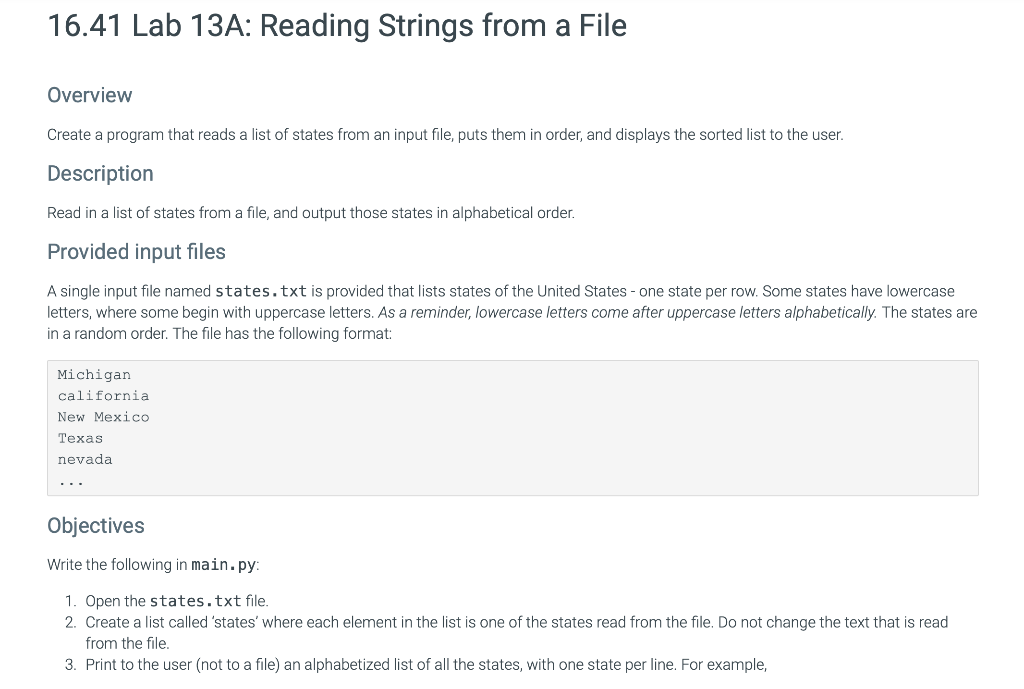The black and white screenshot showcases a web page that presents an assignment labeled "16.41 Lab 13A: Reading Stories from a File". The primary objective of the lab is clearly written in large font at the top, detailing the task of creating a program to read a list of states from an input file, sort them, and display the ordered list to the user.

Below the main title, a smaller font provides the "Overview": "Create a program that reads a list of states from an input file, puts them in order, and displays the sorted list to the user." Further down, under "Description", the task is explained in greater detail: "Read in a list of states from a file, and output those states in alphabetical order."

The input provided is specified as a single file named "states.txt" which includes a list of U.S. states, one per row. It is noted that the states may have varying capitalization, which affects alphabetical sorting since lowercase letters follow uppercase ones.

An example of the file format is shown, with states listed in random order: Michigan, California, New Mexico, Texas, and Nevada.

The "Objectives" section instructs students to perform the following steps in a script named "main.py":
1. Open the "states.txt" file.
2. Create a list called "states", where each element is a state read from the file without altering the text.
3. Print the alphabetically sorted list of states directly to the user, with each state on a new line.

An example output format is also indicated, demonstrating how the user should see the states listed.